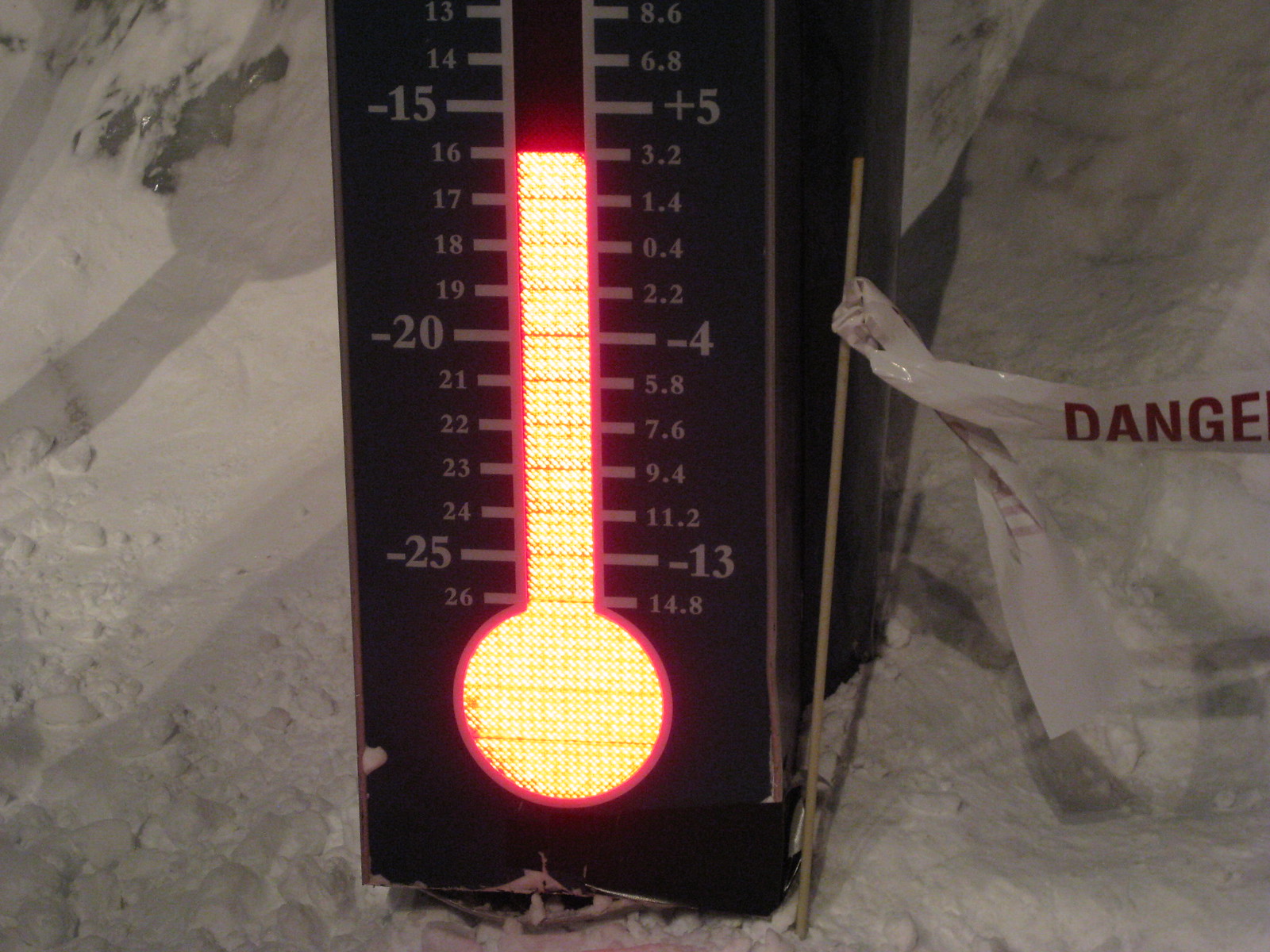An image depicts an electronic outdoor thermometer mounted on a vertical surface, possibly in a mountainous area, as evidenced by the surrounding snow and visible ice. The thermometer displays a reading of 3.2 degrees Celsius. The device is uniquely illuminated, with a bright yellow light filling both the large bulb at the base and the segments of the stem leading up to the current temperature. Nearby, a plastic stick embedded in the ground bears a "Danger" warning, likely indicating hazardous icy conditions. In the foreground, the photographer's shadow is cast, adding a human element to the frosty scene.